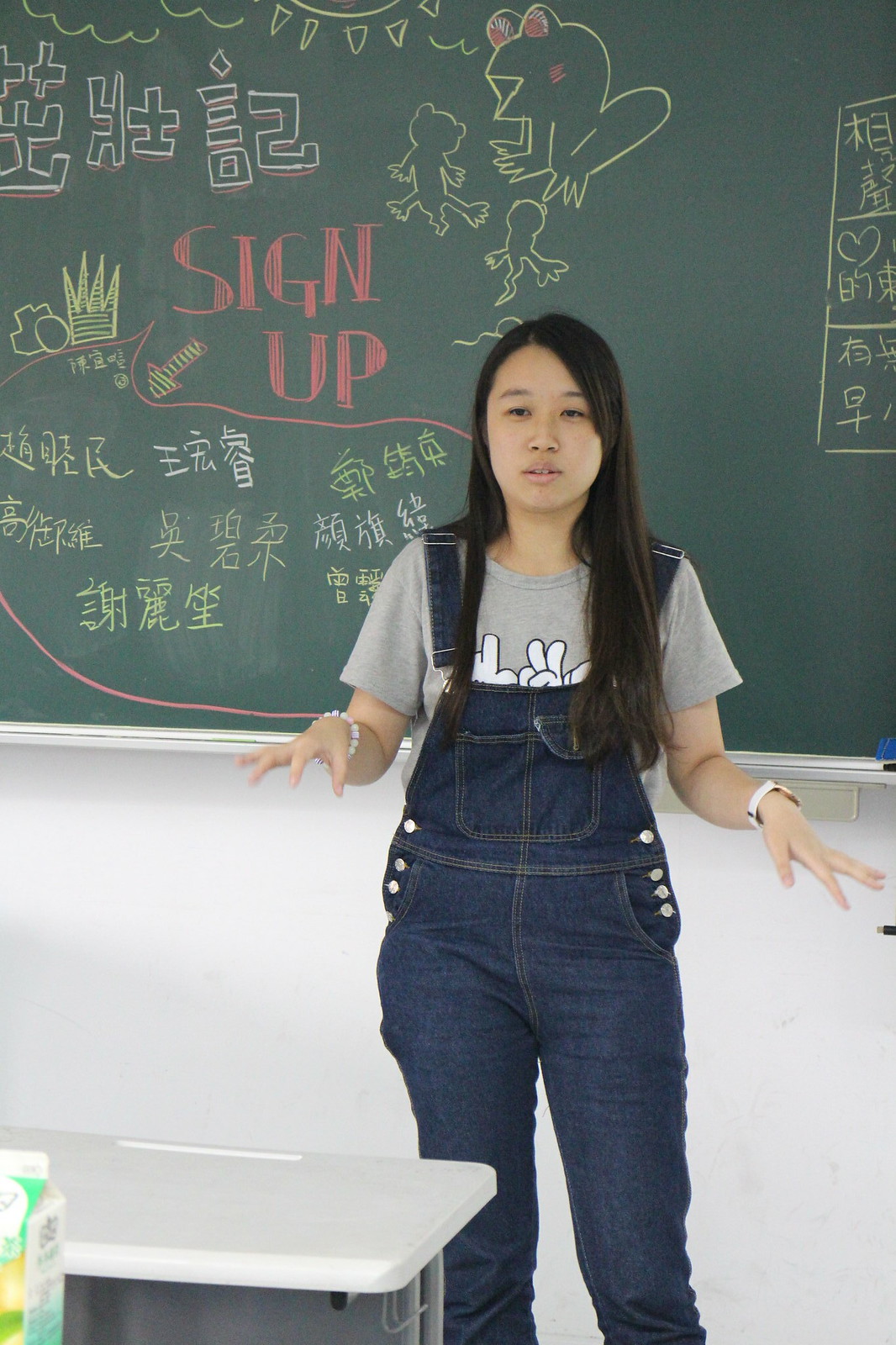In the image, a teenage girl stands facing the camera, positioned in what appears to be a brightly lit classroom. She is wearing overalls over a grey shirt, with a bracelet on one wrist and a watch on the other. Her long hair frames her face as her hands, slightly blurred in motion, suggest she might be teaching or speaking. Behind her, a chalkboard is covered in a mix of Asian characters, possibly Chinese or Japanese, along with colorful drawings such as a frog, clouds, and a partially visible sun. Prominently, the words "sign up" are written in red on the board, adding a distinct contrast to the scene. The vibrant and clear setting shows no other people, highlighting the girl as the central figure in this educational environment.